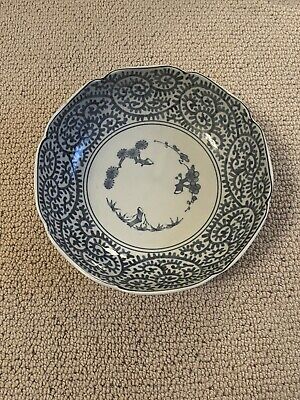This is a photograph of an intricately designed, antique-looking china bowl resting on what appears to be a dense, beige or taupe carpet or possibly a textured tablecloth. The bowl itself is somewhat shallow and has a striking and slightly irregular shape, which could be due to the unique design or perhaps the angle from which the photo was taken. It predominantly features a blue and white color scheme.

The upper rim of the bowl is slightly crimped like a flower and leads down to a large white center circle. Surrounding this center, there are blue swirls and scrolls, possibly representing vines, that extend around the inner part of the bowl. The innermost part of this white center circle features intricate hand-painted designs segmented into threes. These designs include patterns that hint at wreaths, grass-like elements, and possibly flowers, mountains, and berries, although the exact figures are somewhat indistinct and blurry. The bowl is empty, displaying its ornate interior clearly. The craftsmanship suggests it is an antique piece, celebrated for its elaborate and detailed artwork.